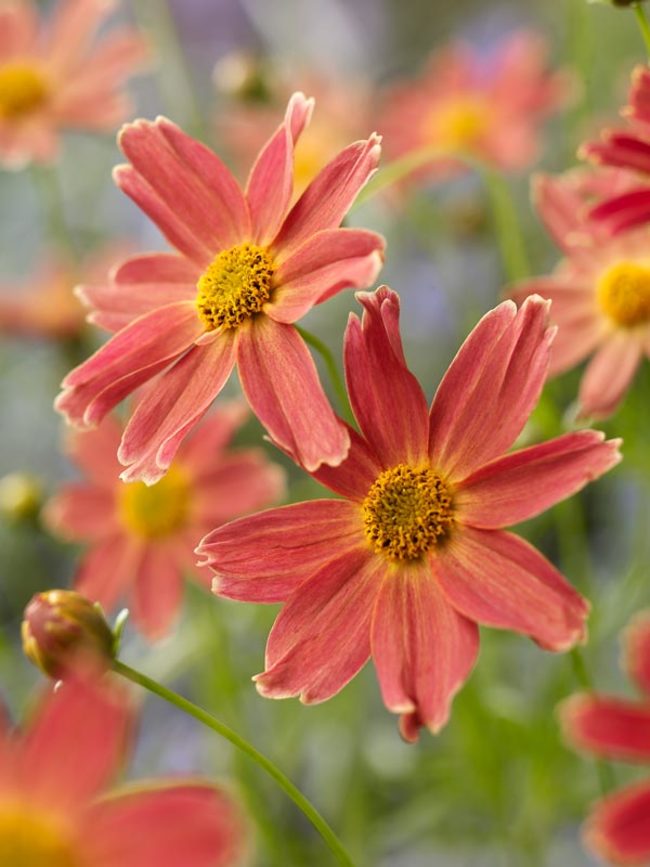This close-up photograph showcases two vibrant flowers at the center of the image, surrounded by several blurred flowers receding into the background. These two central flowers are fully bloomed, with hot pink petals that gradually transition to yellow towards the center, where they encircle a cluster of yellow pollen. Each petal, measuring approximately an inch to an inch and a half in length, is irregular at the tips with subtle white accents. The flowers are supported by slender, vibrant green stems, which also feature some leaves near the base. Notably, on the left side of the image, there is a flower bud yet to bloom. The overall composition, set against a blurry backdrop of green foliage and similar flowers, suggests a lively early spring scene, with an emphasis on the striking contrast between the flowers' rich hues and their surroundings.